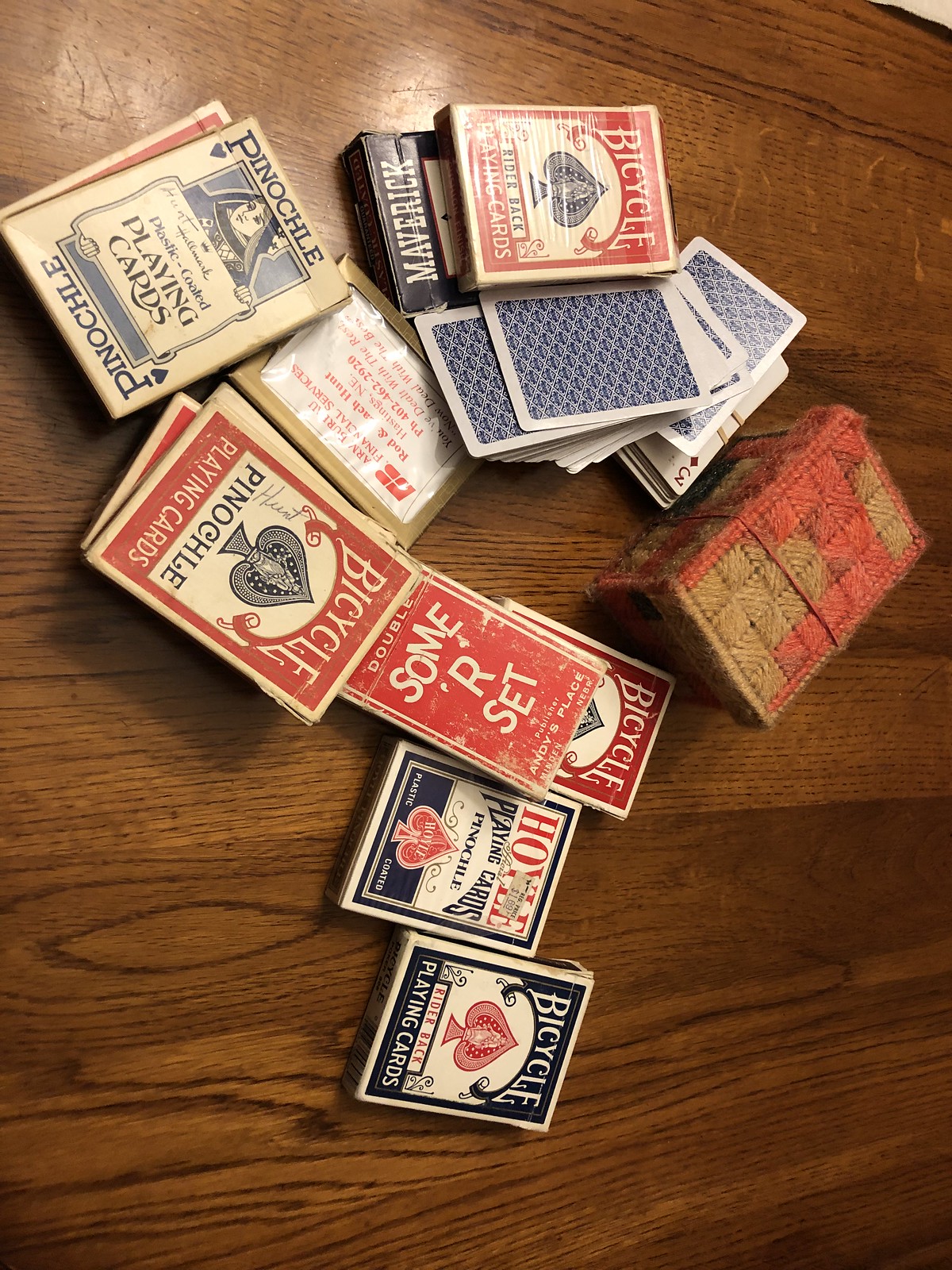An intricately patterned wooden table, showcasing a spectrum of brown hues, serves as the base for an array of playing cards. The table's surface features diverse shades of brown, from light with intricate wood grains to rich, darker areas, creating a visually engaging backdrop. Spread across this wooden expanse are various styles of playing card decks. 

Notably, a couple of Bicycle brand decks, distinguishable by their iconic packaging, catch the eye. One deck is housed in a white box adorned with blue accents and a red spade emblem. Another Bicycle deck in a red box prominently displays "Double Some Are Set" in white print. Additionally, a red "Bicycle Pinochle" deck incorporates a blue spade emblem, indicative of its specialty card type. 

Among these is also a white box labeled "Pinochle Plastic Coated Playing Cards," featuring an image of a woman with a blue veil. Besides the boxed decks, an array of loose blue and white patterned cards lie neatly stacked. To complete the spread, a fabric-knit style box, secured with a rubber band, likely serves as protective storage for one of the card decks.

The detailed array of cards and their packaging against the multihued wooden table creates a captivating scene, inviting observers into a world of classic card games.